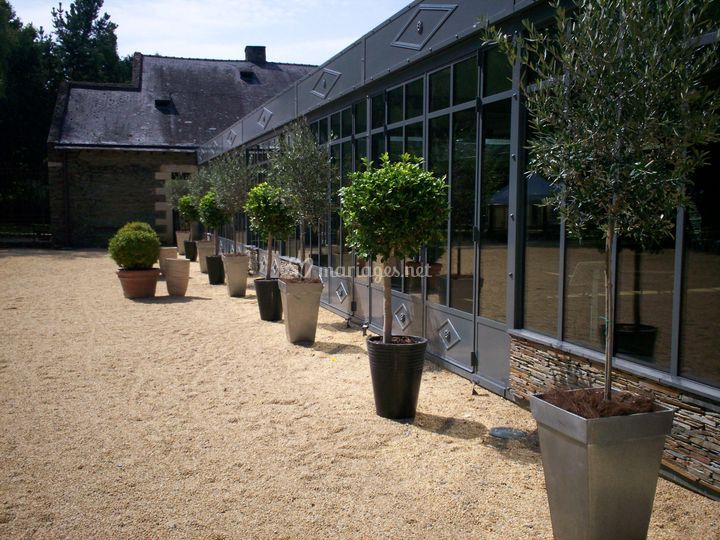The image features the exterior of a single-story, horizontal, rectangular black building, characterized by numerous vertical glass windows with metal frames and a stone facade along its base. The surface outside the building is covered with light tan, sandy dirt or gravel. Arranged diagonally from the lower right-hand corner towards the middle left are various potted plants, predominantly small trees and bushes. These plants are contained in a mix of tall, conical black pots and gray square pots that taper wider towards the top, with some white circular planters visible as well. In the background, there's a brick house with a black roof and a prominent chimney, along with dense green trees in the upper corners of the image. Above it all, the sky is a light blue with faint white clouds. The entire scene is subtly watermarked with a heart and the text “marriages.net” overlaying the image.